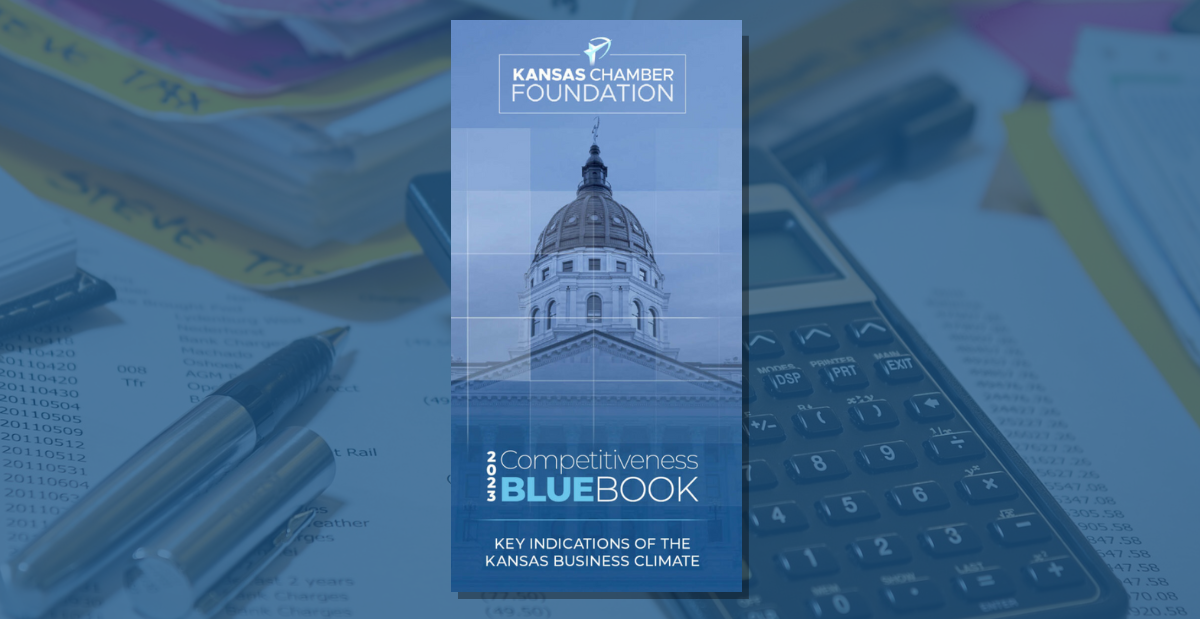The image features a blue pamphlet prominently centered, set against a slightly faded, darkened background of office materials. The pamphlet showcases a picture of a Capitol building with "Kansas Chamber Foundation" written at the top in white text within a white square. Below the Capitol building image, the text reads "2023 Competitiveness Blue Book," with "Blue Book" highlighted in light blue, and beneath a dividing line, it states "Key Indications of the Kansas Business Climate." An abstract logo resembling an archer is also present near the top. The pamphlet casts a subtle drop shadow to the right. Surrounding the pamphlet, the background features a clutter of office supplies including a calculator, scattered pens, sticky notes, and a yellow folder brimming with papers, as well as various charts and documents strewn across the desk.